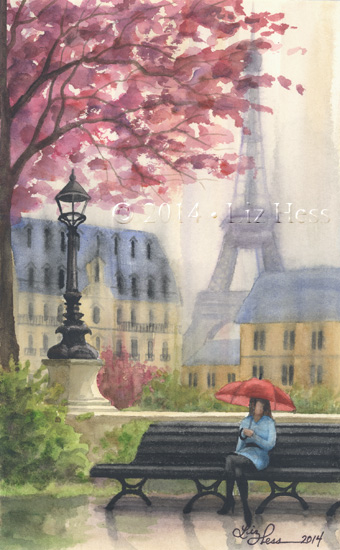This rectangular watercolor painting, approximately 4 inches high and 2.5 inches wide, depicts a Parisian scene with the iconic Eiffel Tower dominating the background. At the forefront, a woman sits on a black bench, holding a vibrant pink umbrella that contrasts with her long-sleeved blue dress and black leggings. Her face lacks detail, as the artist has chosen not to represent her facial features. The woman's outfit is complemented by her dark brown hair and black shoes. To the left of her, a large tree with striking pink and red leaves stretches up to the top of the painting. A green bush and a low stone fence are also present, with a black streetlamp perched on the fence beside her. Behind the woman, under the shadow of the Eiffel Tower, stand several large buildings. The artist's signature, "Liz Hess, 2014", is inscribed in black cursive in the lower right-hand corner.